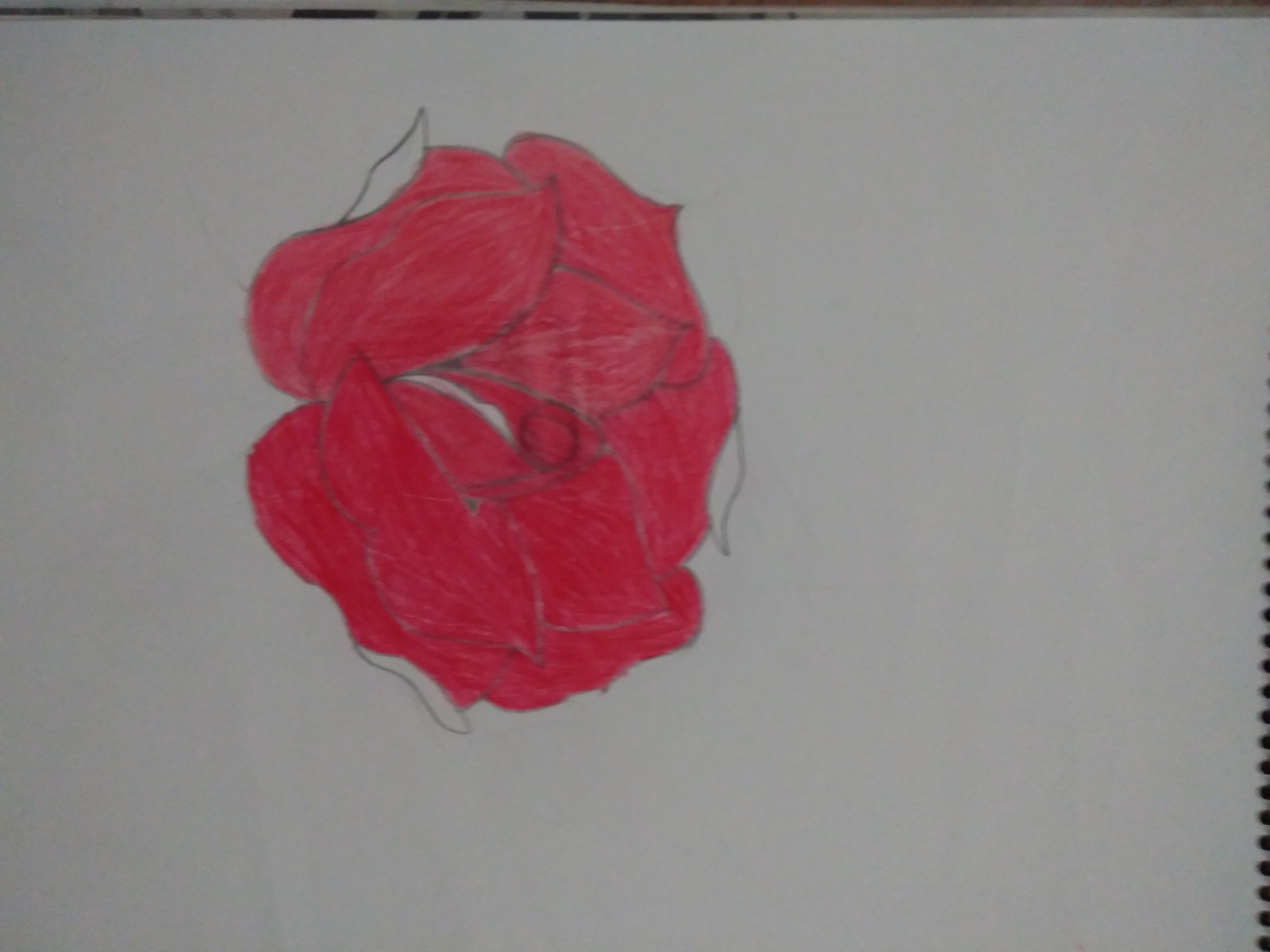This is a detailed drawing of a flower, likely a rose, rendered on white paper that appears light gray. The primary color used is a bright red, applied in what seems to be either colored pencil, fine-pointed marker, or crayon. The flower, occupying roughly 15-20% of the page, is situated off-center towards the upper left part of the paper and oriented slightly downward to the right. The intricate details of the petals are somewhat obscured due to the dense and precise coloring within dark gray graphite pencil outlines. These petals exhibit a pattern of coming to a point before curving back inward, with an estimated four or five petals per layer. There's a round center, showing a noticeable white streak arcing towards the upper left corner, giving the flower a folded appearance. Additionally, three uncolored leaves outlined in gray graphite surround the bloom. The presence of a perforated edge on the right side, visible from about two-thirds down, suggests that the drawing is part of a spiral-bound sketchbook.